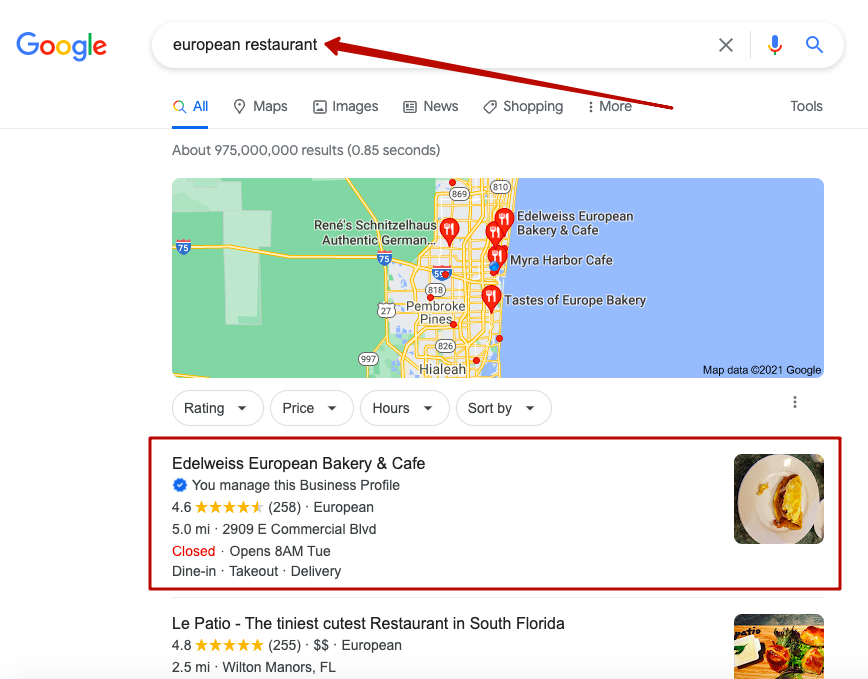The image captures a Google search results page focused on "European restaurant." The backdrop is a clean white, featuring the iconic multicolored Google logo in the upper left corner. To its right, a long rectangular search box with rounded edges displays the search query "european restaurant" in black lowercase text. Adjacent to the text on the right are a gray "X," a multicolored microphone icon in shades of blue, red, yellow, and green, and a blue magnifying glass icon.

A prominent red arrow overlays the page diagonally, pointing directly at the search term "european restaurant." Directly below, a series of navigation tabs stretch horizontally. The first tab, highlighted in blue with an underline, reads "All" and features a multicolored magnifying glass icon. Next are tabs labeled "Maps," "Images," "News," "Shopping," and "More," each accompanied by relevant icons. To the far right is a tab labeled "Tools."

Beneath the tab line, gray text indicates "About 975,000 results (0.85 seconds)." A small segment of a Google Map is displayed below, marked with business names in black text. Notable locations include "Rene's Schnitzelhaus (Authentic German)," "Eidelweiss European Bakery and Cafe," "Myra Harbor Cafe," and "Taste of Europe Bakery."

Following the map are four dropdown tabs labeled "Rating," "Price," "Hours," and "Sort By." Featured prominently beneath these dropdowns is information about "Eidelweiss European Bakery and Cafe." Details include a blue and white check mark indicating business management, five gold stars, a rating of "4.6 (250)," and descriptors such as "European," "5.0 MI," and the address "2909 E Commercial BLVD." The café's status is noted in red text as "Closed," with additional operational details indicating it opens at 8 a.m. for dine-in, takeout, and delivery. An accompanying image features a white dinner plate with yellow food. This section is bordered by a bright red rectangle.

Just below is information for "La Patio: The Tiniest Cutest Restaurant in South Florida," featuring a rating of "4.8" alongside five gold stars, and in brackets, "(255)." Additional descriptors include "European," a distance of "2.5 MI," and the location "Wilton Manors, Florida." The associated image displays a wooden chopping board topped with three browned pieces of food served on a green garnish.

This intricate layout provides a detailed snapshot of the search results page, highlighting various elements from text and tabs to visual markers and business specifics.